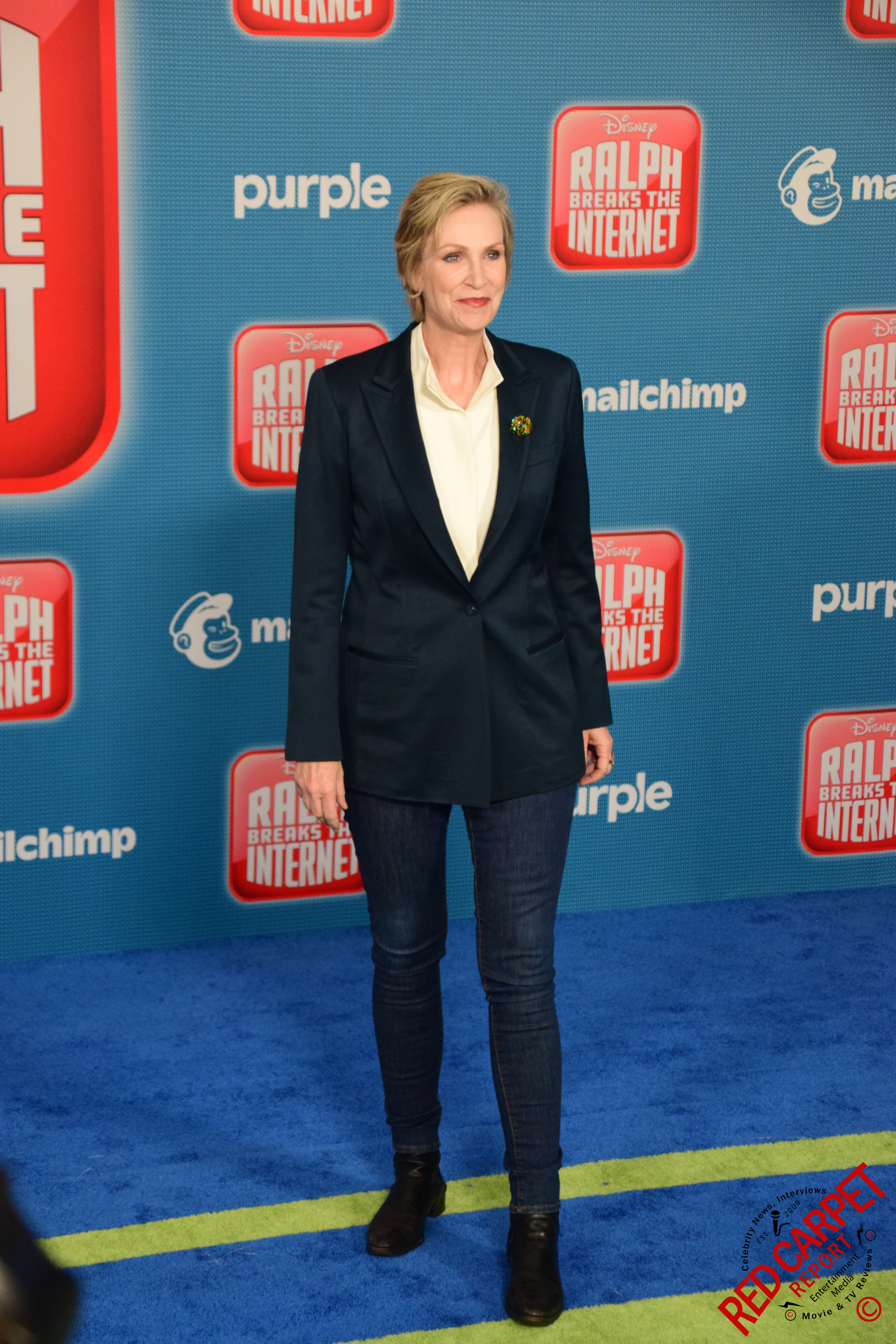In this photograph, a distinguished actress, likely in her 40s or 50s, stands confidently at a red carpet event for the Disney film "Ralph Breaks the Internet." She is poised in front of a light blue backdrop adorned with various logos, including the most prominent red rectangle that reads "Disney Ralph Breaks the Internet" in white text. Notably, there are also white text logos for "Purple" and "MailChimp," the latter accompanied by a profile of a cartoon monkey. The watermark "Red Carpet Report" is visible in red text in the bottom right corner of the photograph.

The actress stands on a predominantly blue carpet, accented with greenish-gold stripes, complementing her attire. She wears tight-fitting blue jeans paired with black ankle boots, and a professional black sports coat buttoned over a yellowish-white button-up shirt with an open collar. Her short blonde hair and earrings enhance her polished and attractive appearance as she gazes toward the camera, ensuring her presence is unmistakable at this premiere event.